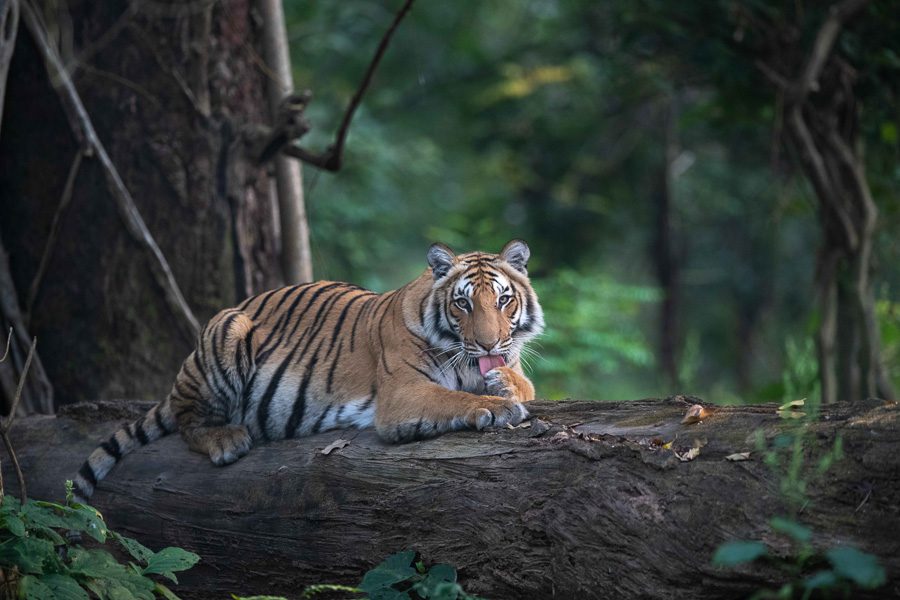This detailed real-life photo captures a majestic tiger resting in its natural jungle habitat. The horizontal rectangular image showcases a vibrant scene of a dense, dark green forest with a blurry background of trees, plants, and shrubs. The tiger, with a soft light orange or brown coat adorned with black stripes and white underbelly, is laying on a broad tree trunk that has fallen and stretches horizontally across the frame. The tree trunk is a dark grayish-brown color, blending with the lush surroundings. To the left of the tiger, another tree trunk stands vertically, adding depth to the scene.

The tiger's positioning on the trunk is somewhat low to the ground, indicating the tree has fallen or is heavily leaning. The imposing big cat is facing the camera directly, creating an intense and captivating gaze. Its head is framed with a mix of white and black fur around the eyes and nose, highlighting its menacing yet magnificent expression. The tiger's mouth is slightly open as it licks its paw, displaying its pink tongue. The overall composition of greens and browns creates a vivid contrast with the tiger's striking appearance, making it the focal point of this awe-inspiring wildlife photograph.